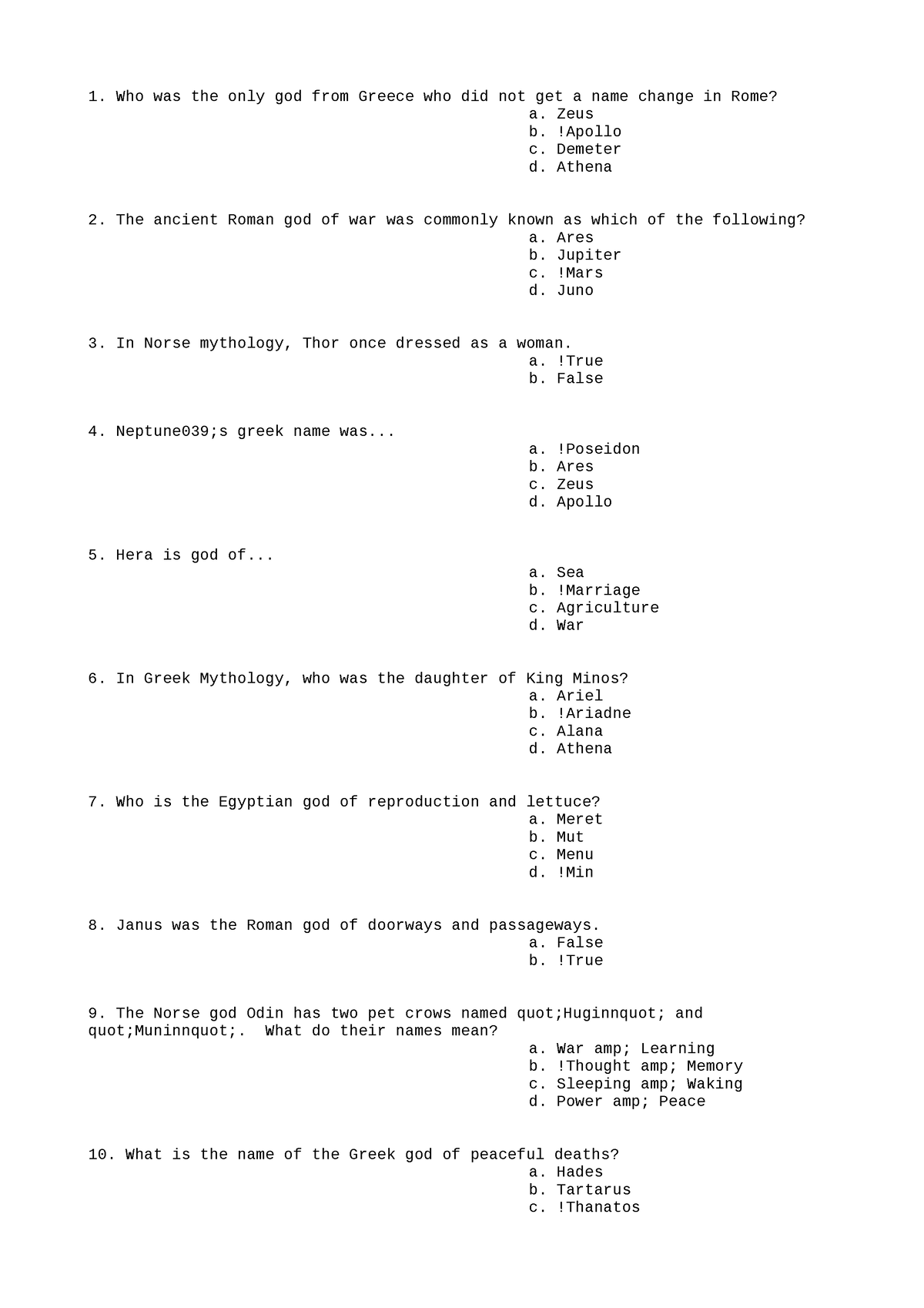The image displays a detailed chart structured as a test questionnaire. The chart is organized into one long column featuring ten questions, each designed to evaluate knowledge on mythological figures. The questions are accompanied by multiple-choice answers, with certain choices highlighted to indicate correct answers. Below is a detailed breakdown of the questionnaire:

1. **Question 1: (Top left)**
   - **Question:** Who was the only Greek god who did not get a name change in Rome?
   - **Options:** Zeus, Apollo, Demeter, Athena
   - **Correct Answer:** Apollo (marked with an exclamation mark)

2. **Question 2:**
   - **Question:** The ancient Roman god of war was commonly known as which of the following?
   - **Options:** Aries, Jupiter, Mars, Juno
   - **Correct Answer:** Mars (marked with an exclamation mark)

3. **Question 3:**
   - **Question:** In Norse mythology, Thor once dressed as a woman. True or false?
   - **Options:** True, False
   - **Correct Answer:** True (marked with an exclamation mark)

4. **Question 4:**
   - **Question:** Neptune's Greek name was Poseidon, Aries, Zeus, or Apollo?
   - **Options:** Poseidon, Aries, Zeus, Apollo
   - **Correct Answer:** Poseidon (marked with an exclamation mark)

5. **Question 5:**
   - **Question:** Hera is the god of sea, marriage, agriculture, or war?
   - **Options:** Sea, Marriage, Agriculture, War
   - **Correct Answer:** Marriage (marked with an exclamation mark)

6. **Question 6:**
   - **Question:** In Greek mythology, who was the daughter of King Minos?
   - **Options:** Ariel, Adriana, Alana, Ariadne
   - **Correct Answer:** Ariadne (marked with an exclamation mark)

7. **Question 7:**
   - **Question:** Who is the Egyptian god of reproduction and lettuce?
   - **Options:** Merit, Mut, Menu, Min
   - **Correct Answer:** Min (marked with an exclamation mark)

8. **Question 8:**
   - **Question:** Janus was the Roman god of doorways and passages. True or false?
   - **Options:** False, True
   - **Correct Answer:** True (marked with an exclamation mark)

9. **Question 9:**
   - **Question:** The Norse god Odin has two pet crows named Hugin and Munin. What do their names mean?
   - **Options:** War & learning, Thought & memory, Sleeping & waking, Power & peace
   - **Correct Answer:** Thought & memory (marked with an exclamation mark)

10. **Question 10:**
    - **Question:** What is the name of the Greek god of peaceful deaths?
    - **Options:** Hades, Tartarus, Thanatos
    - **Correct Answer:** Thanatos (marked with an exclamation mark)

This detailed breakdown emphasizes the structure and content of the quiz, clarifying the questions and highlighting the correct answers for clarity.